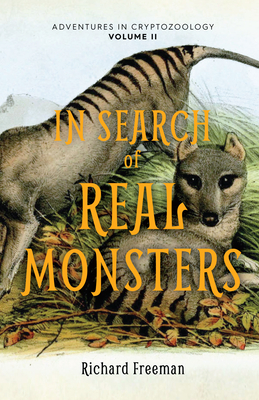The image is a book cover for "Adventures in Cryptozoology, Volume 2" with a white background. The title "In Search of Real Monsters" is prominently displayed in large yellow text across the center. At the top, the series title "Adventures in Cryptozoology" is written in gray, while "Volume 2" appears in black. At the bottom, the author’s name, Richard Freeman, is shown in smaller text.

The illustration features two mysterious, tiger-striped animals. One animal is lying in the grass, displaying a mix of gray and brown fur, reminiscent of a fox with distinct black stripes down its back. The second animal, of a similar appearance, stands behind it, reaching upwards as if stretching or grasping for something. The animals have black eyes, small whiskers, and brown noses. The scene is complemented by green grass, red and green leaves, and twig-like branches, enhancing the natural setting depicted on the cover.